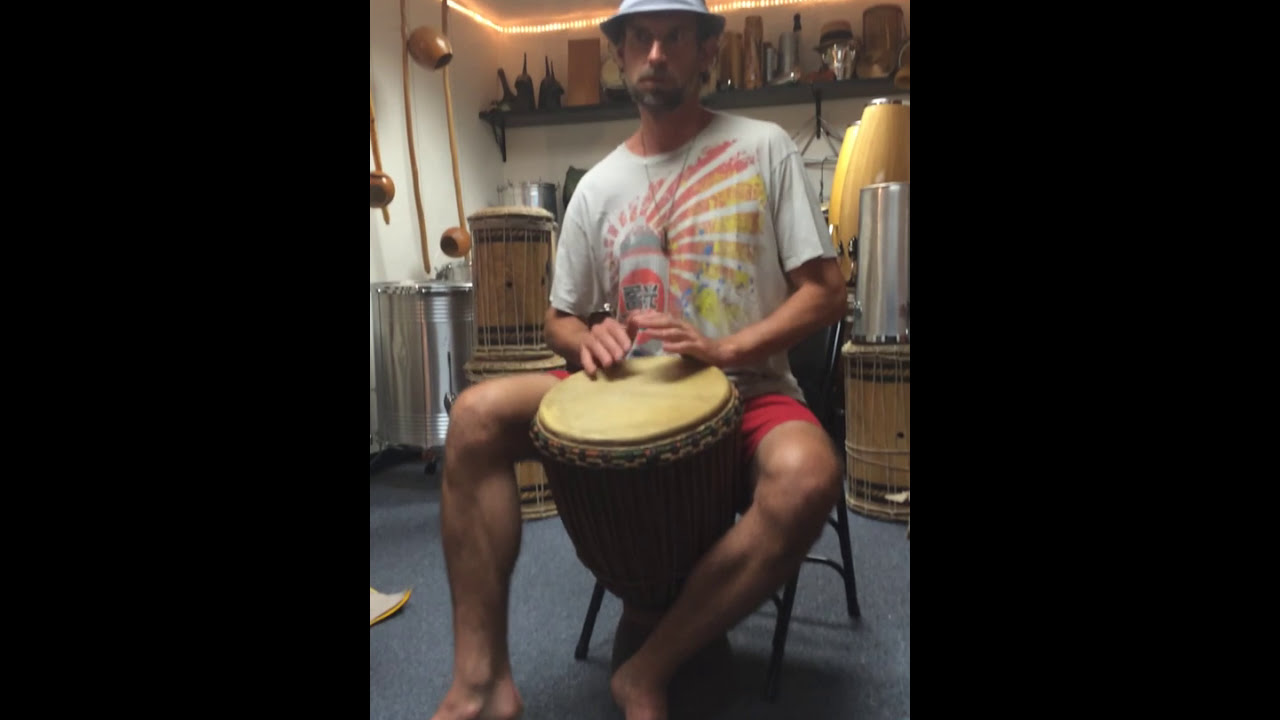In the center of the image, a young man, likely in his 30s, is sitting on a folding chair, facing the camera. He is wearing a blue hat, a white t-shirt adorned with a colorful sunburst design incorporating red, yellow, and orange hues, and red shorts. The man has a beard and mustache, and his face is turned slightly to his right with a straight expression. His hands are poised over a tan and brown djembe drum placed between his legs, suggesting he is playing it. 

Behind him, the scene is filled with various musical instruments and objects. To his left (viewer’s right), there are several drums stacked on top of each other, with a silver drum positioned to the left of the stack. Small wooden drums hang from the wall by ropes, and another set of stacked drums mirrors the arrangement on his right (viewer’s left). Additional shelves in the background hold a mix of drums and various objects, possibly indicating that the man is in a store. The walls are adorned with what appear to be round, brown light fixtures. The image is bordered by a thick black rectangle on the left and right sides, framing the centered composition.